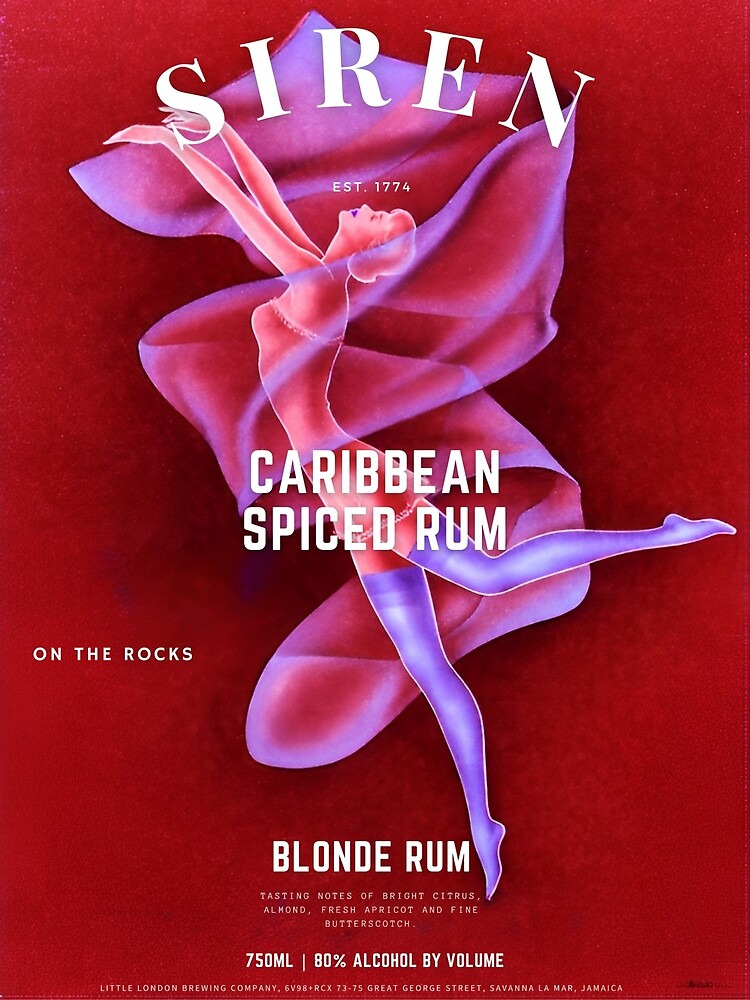This striking red poster showcases Siren Caribbean Spiced Rum, established in 1774 and produced by Little London Brewing Company in Jamaica. The central figure is an illustrated woman, portrayed in a whimsical, almost caricature-like style. She is enveloped in a pink and red ribbon, accentuating her long, extended legs in vivid purple stockings. Her delicate ballerina-style outfit is skimpily designed to cover just above her breasts and just below her buttocks, contributing to her ethereal appearance. With arms gracefully extended and head tilted back, her blonde hair and purple lips add to the mystique. The bold white letters at the top spell "Siren," with "Blonde Rum" and tasting notes of bright citrus, almond, fresh apricot, and fine butterscotch featured prominently. Below, it specifies "80% alcohol by volume" and "750 milliliters," emphasizing the potency of the rum. The detailed illustration and the luxurious descriptions make this poster an enticing advertisement for rum connoisseurs.